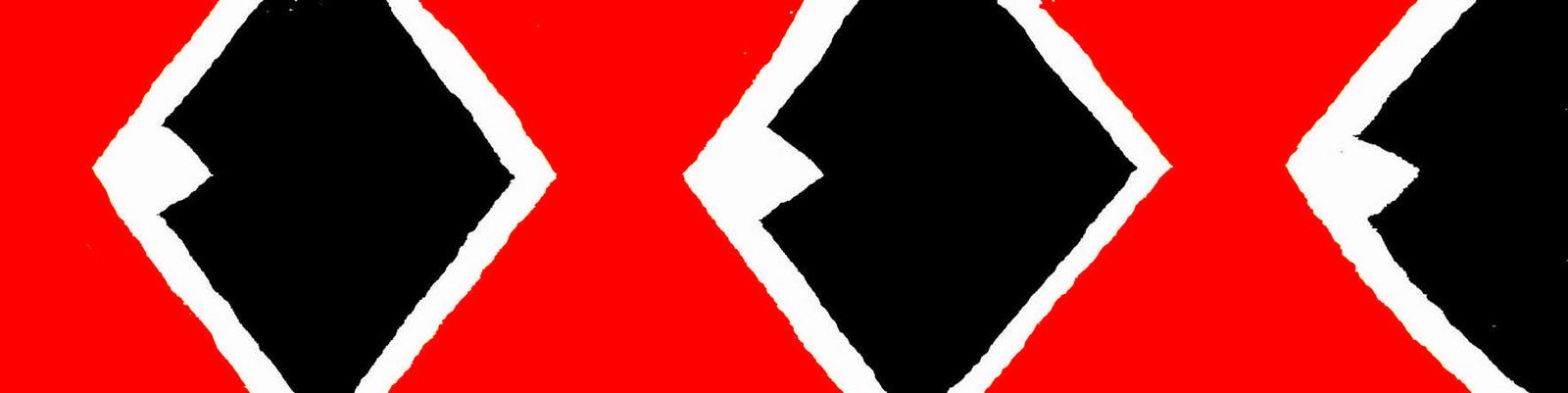This painting features a vibrant, rectangular red background with three prominently placed, rhombus-shaped designs. Each rhombus has a white border with a smaller black rhombus enclosed within it. Notably, the leftmost rhombus is cut in half, creating a triangular white section where the black is absent. Similarly, the third rhombus on the right is also cut in half, resulting in a partial visible shape. The central rhombus remains intact, showcasing the full contrasting colors. The overall composition is simple yet striking, with the angular placement of the rhombuses adding a dynamic element to the artwork.